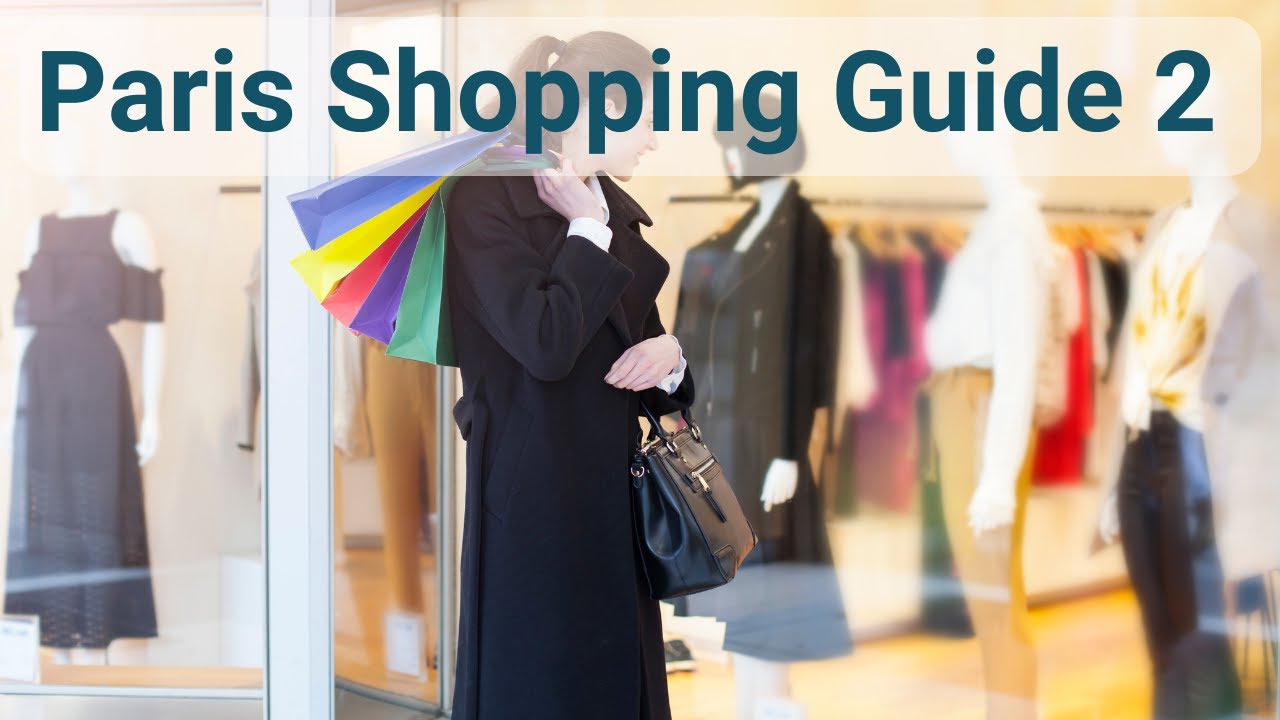A rectangular advertisement banner at the top of the image reads "Paris Shopping Guide 2" in dark green text. The central figure is a woman with long hair tied in a ponytail, seen from the side with her face turned to the right. She is dressed in a black wool jacket over a white shirt and carries a black purse with a zipper. Over her left shoulder, she holds several colorful shopping bags in blue, yellow, red, purple, and green. The background reveals a store window displaying various mannequins dressed in different outfits: a beige pants and white shirt ensemble, a white shirt and black pants combination, a mannequin in a wool jacket, and another in a black dress. Additionally, there is a rack of clothes blurry but discernible in the store's interior.